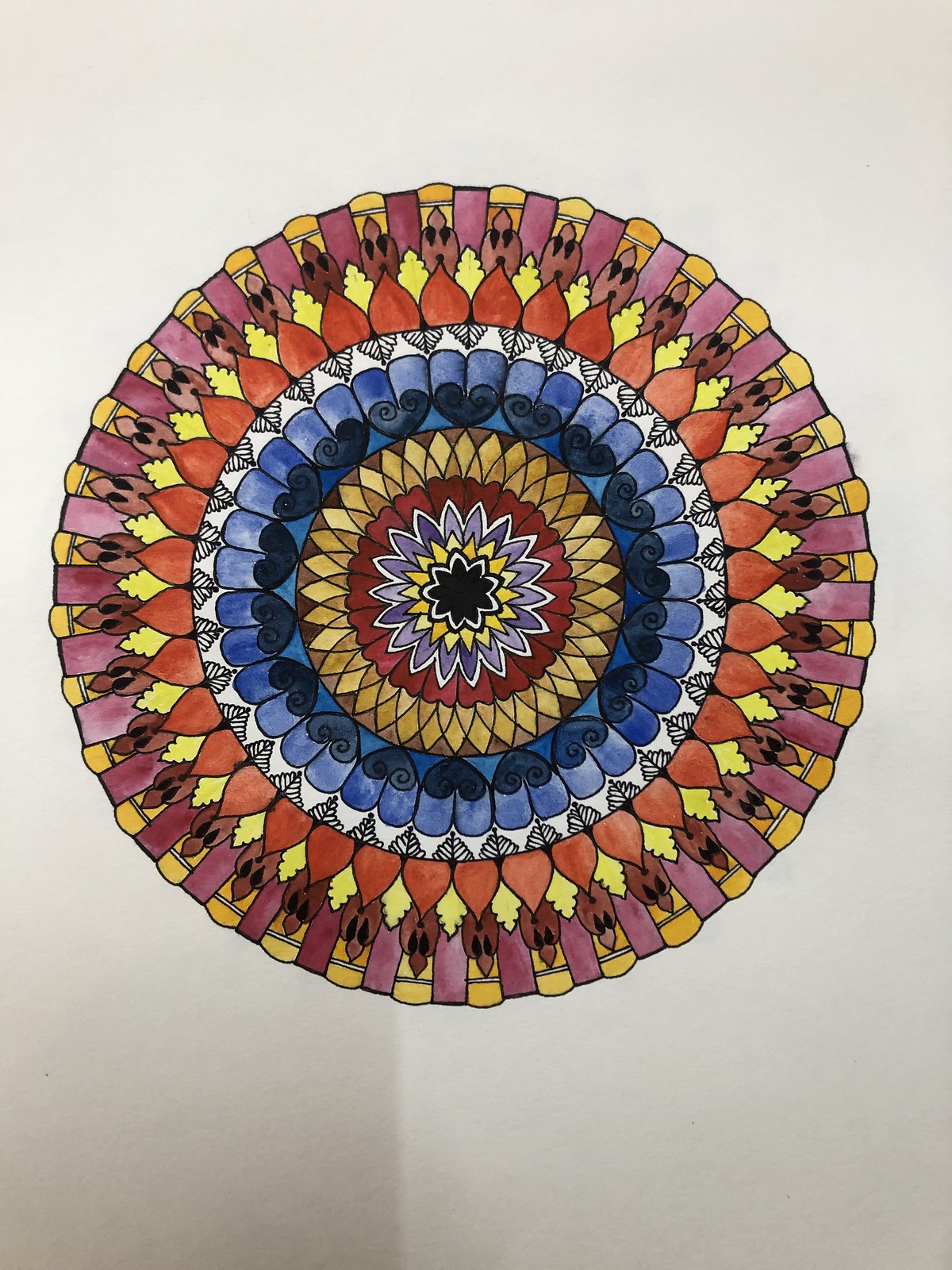This image depicts a highly detailed, circular, abstract piece of art that is rich with vibrant and varied colors, resembling a layered design similar to the rings of a tree trunk or the intricate patterns of a stained glass window. It features a central motif that starts with a black star or flower shape, surrounded by a white outline. Moving outward, the design incorporates layers of yellow petals, light purple petals, dark red circles, and light brown petals. It then transitions into layers of dark purple hearts with lighter purple hearts and white sections that have light purple leaves. The outer layers showcase blue heart shapes, orangish-red flower petal shapes, purple rectangles, and small purple stripes. The background appears to be a light gray, possibly a folded sheet of paper, enhancing the intricate patterns and detailed craftsmanship of what seems to be a beautifully braided rug or a meticulous knit piece.